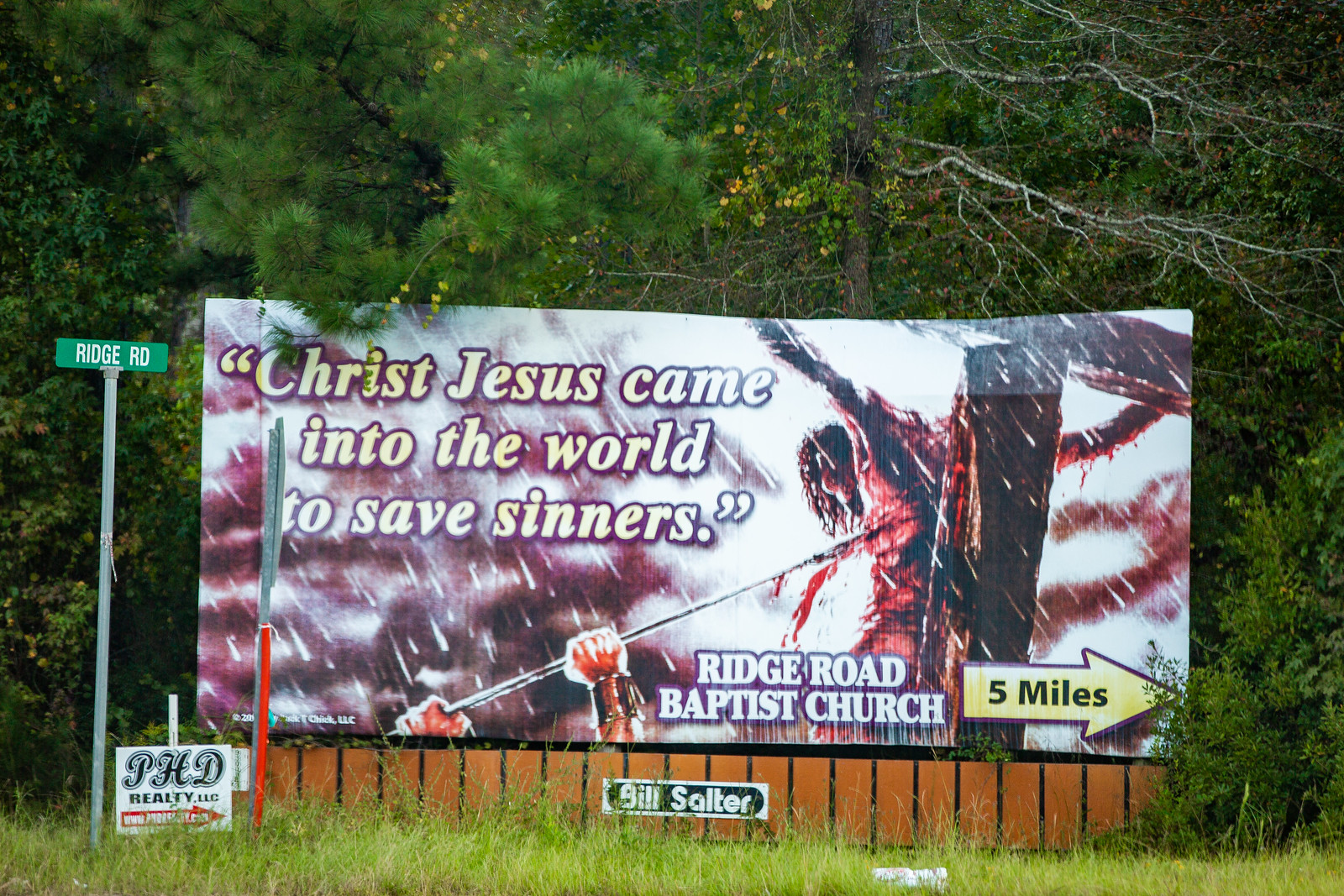This photograph captures a vivid and striking outdoor scene during the day. On the left side, a green street sign with white capital letters reads “RIDGE ROAD.” Below, there is a verdant expanse of grass, and various species of trees populate the background, creating a lush setting.

Adjacent to the Ridge Road sign is a blue real estate sign for “PhD Realty Inc.” The text “PhD” is written in cursive, accompanied by a red arrow pointing toward additional text. Nearby, there is a stop sign noticeable by the red strip on its side.

Dominating the right side of the image is a prominent billboard with a powerful religious message. The billboard displays the quote, “Christ Jesus came into the world to save sinners,” alongside “Ridge Road Baptist Church.” A yellow arrow beneath this text points to the right, indicating that the church is five miles away. 

The central illustration of the billboard is both dramatic and poignant. It depicts Jesus on the cross, with a Roman soldier's hand reaching up from below. The hand, identifiable by a gladiator arm band, wields a pike that pierces Jesus’s side, causing blood to spurt out. The red splatters merge with the clouds, giving the impression that they are also stained. Below this illustration, the name “Bill Salter” appears twice, suggesting he is the creator of the sign.

The overall composition of the image intertwines religious symbolism, local signage, and natural elements, presenting a multi-faceted and intense visual narrative.